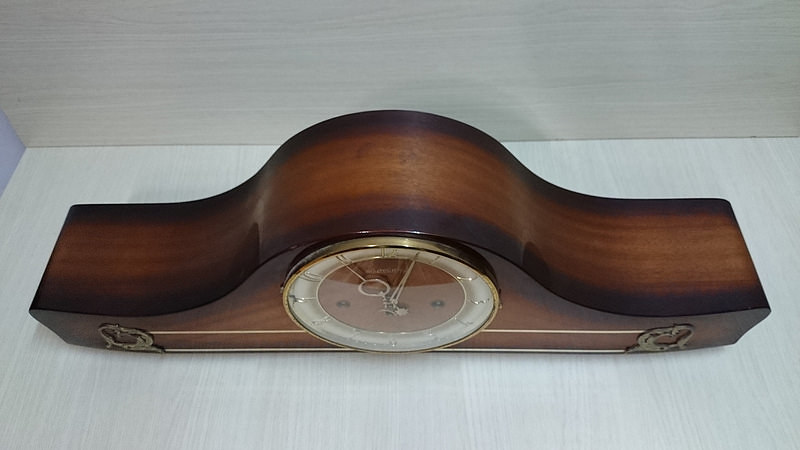The photograph showcases a vintage mantle clock viewed from the front and above, resting on a light beige wood surface. The clock's body is constructed from richly polished mahogany wood, darkening at the edges and illuminating a distinctive central strip. The overall shape of the clock resembles a sleigh or a pirate's hat, with a flat bottom and delicately curved sides that swoop upwards to form an elegant arch over the central, round clock face.

This clock face, positioned at the peak of the wooden arch, features a white ring where Roman numerals are mounted, surrounding a brown center. The golden hour and minute hands stand out prominently against this background. Decorative brass or gold metal pieces in floral or leaf patterns adorn the left and right sides of the clock's front, connected by subtle gold horizontal lines that stretch across the wooden surface. The combination of dark mahogany and golden accents creates a striking, timeless aesthetic indicative of a classic vintage design, perfect for display on a mantle or above a fireplace.